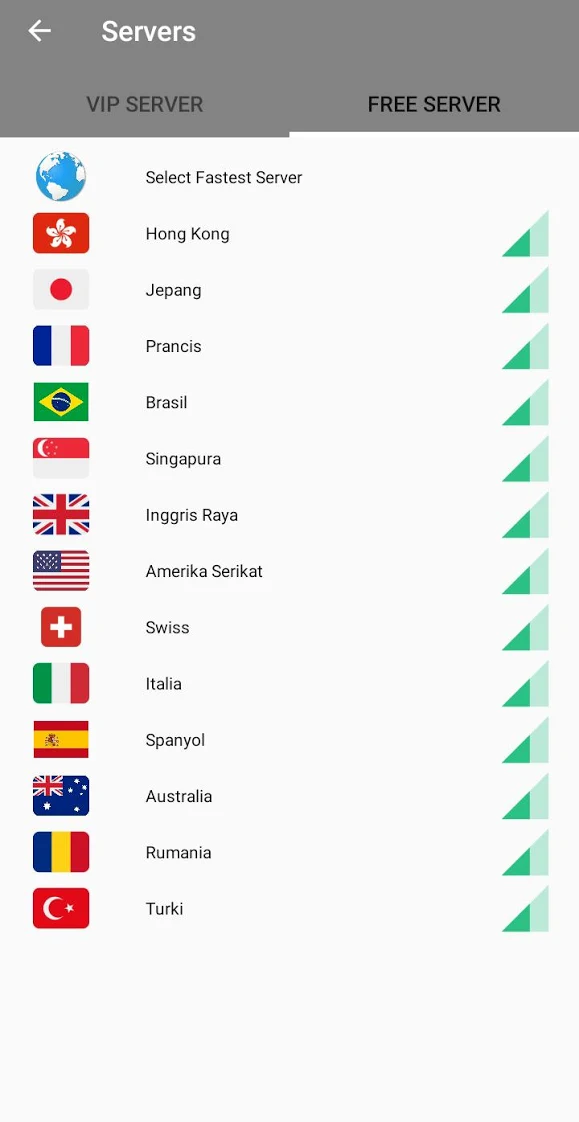The image displays a grey stripe running horizontally across the top with a left-pointing arrow located in the upper left corner, labeled "Servers" below it in black text. On the left side of the stripe, it says "VIP Server," and on the right side, it says "Free Server," with the selection toggled to the "Free Server."

Beneath the grey stripe, the background transitions to white, featuring a globe icon on the left. The text is left-aligned, starting with the heading "Select Fastest Server." Listed below are various country names, each preceded by its national flag. The countries listed are:

- Hong Kong
- Japan (miswritten as "Jpang")
- France (miswritten as "Francis" and "Prancis")
- Brazil
- Singapore (misspelled)
- United Kingdom (with its Union Jack flag, referred to as "British flag")
- United States (miswritten as "Americas Serikat")
- Switzerland
- Italy (written as "Italia")
- Spain (miswritten as "Spagnola")
- Australia
- Romania (miswritten as "Rumania")
- Turkey (miswritten as "Turki")

Each country has a green rectangle bar to the right, indicating the status or quality of the server connection.